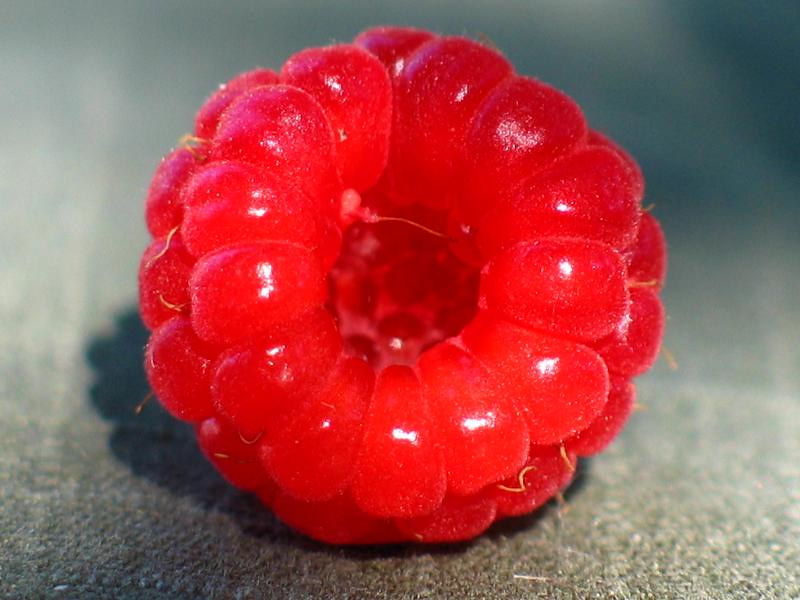The image showcases an extreme close-up of a single vibrant red raspberry, which takes up almost the entire frame. The intricate details of the raspberry are clearly visible, including the tiny, hair-like structures on the surface and the multitude of small, round drupelets that make up the berry. The raspberry is lying on its side, exposing the hole at the top, and you can see the shorter, narrower inner ring and the wider outer ring. The raspberry is resting on a textured gray cloth, possibly denim or canvas, with a faint plaid pattern, suggesting it might be on someone's lap. The cloth appears rough, with visible white lines and a noticeable shadow cast by the raspberry. The foreground of the image, including the raspberry's detail and the cloth's texture, is sharply in focus, while the background fades into a blur, enhancing the overall aesthetic of the image and its minimalistic beauty.